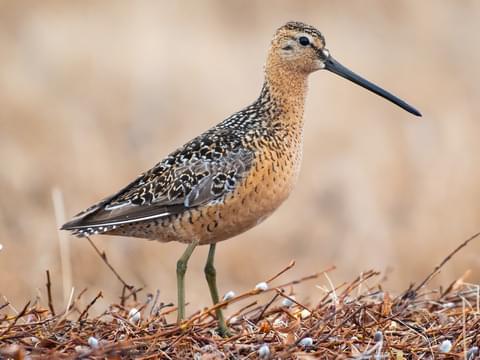This detailed close-up photo captures a bird with a remarkably long and thin black beak. The bird’s head and chest are predominantly brownish-tan, transitioning to a mix of gray, black, and white across its wings and back. Its legs are spindly and have a greenish-gray hue. The bird's eyes are black and it is facing to the right, standing on what appears to be the edge of a nest-like structure composed of tightly interwoven twigs. Some of the twigs have small, white buds which add texture to the scene. The background is blurred and displays an indistinct mix of tan, gray, and white, suggesting an outdoor, nature-filled environment with potentially grassy and earthy tones. The daylit setting enhances the natural ambiance of this intriguing portrait.